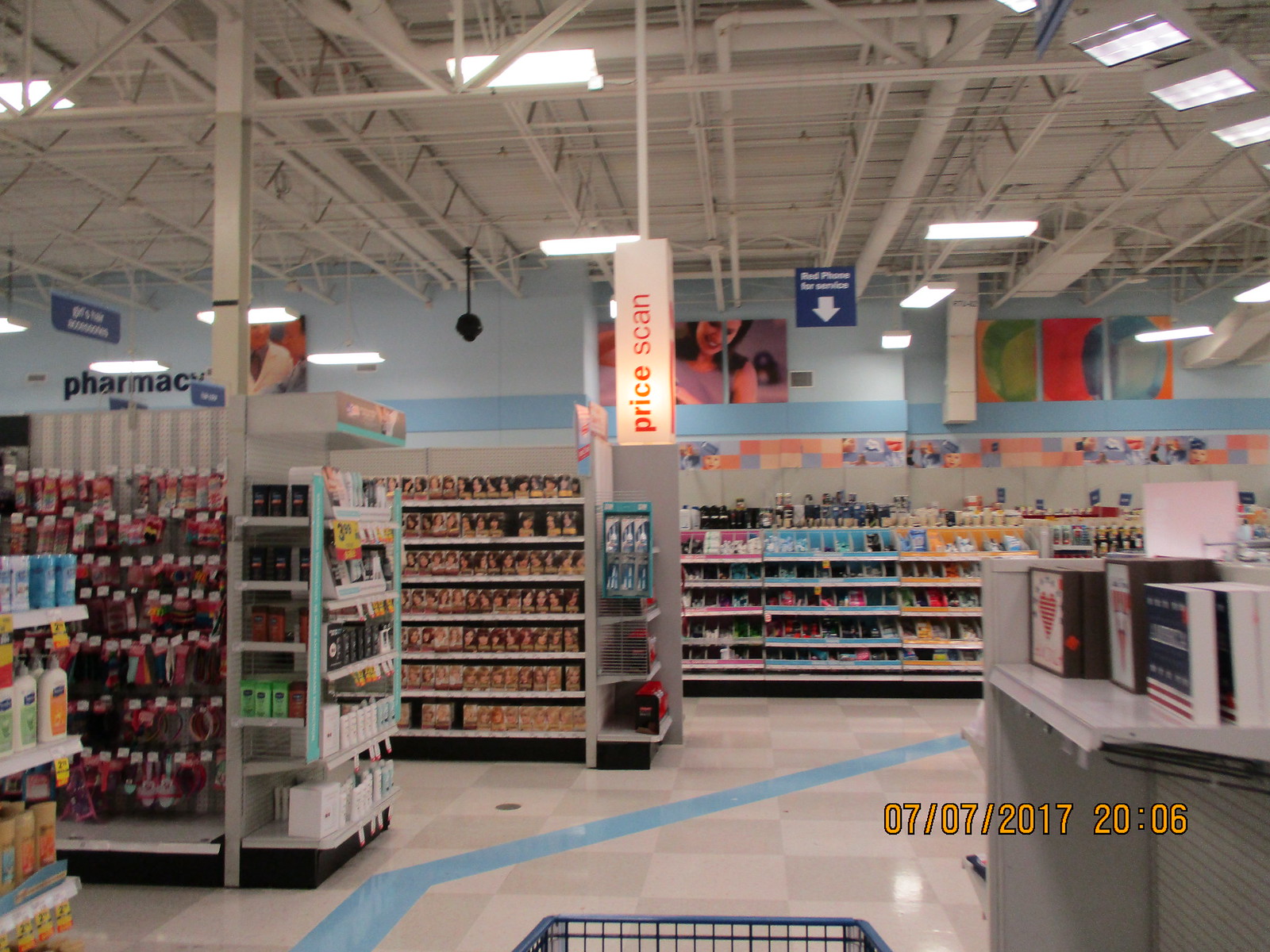The image captures a well-lit, high-quality, color photograph of the interior of a sizeable retail store, possibly a pharmacy like CVS, taken on July 7, 2017, at 20:06. The scene features a date and time stamp in yellow numbers at the lower right corner. Prominently visible in the photograph are several aisles stocked with various products. On the extreme left side, you can see shelves displaying what appear to be lotions or sunscreen products. Next to that, there's an aisle filled with hair color boxes, identifiable by the faces of women on the packaging.

Further into the image, a white sign with vertical orange letters saying "Price Scan" is hanging from the ceiling atop a post. This self-service price scanner is illuminated and stands out clearly. Back towards the left center of the image, black lowercase letters on the back wall spell out "pharmacy," indicating the location of the pharmacy section of the store.

Lower shelves run along the back wall with colorful displays in purple, blue, and orange, though their contents are not immediately discernible. To the right side of the photo, there is a counter or customer service desk laden with objects that appear to be books or signs. In the bottom edge of the image, the front portion of a blue wire shopping cart peeks into view, suggesting the perspective of a shopper navigating the store.

The store features a highly polished beige and white checkerboard floor pattern with a light blue stripe marking the main walkways. The ceiling is notably high, exposing metal frame rafters that add a structural, industrial vibe to the store's interior.